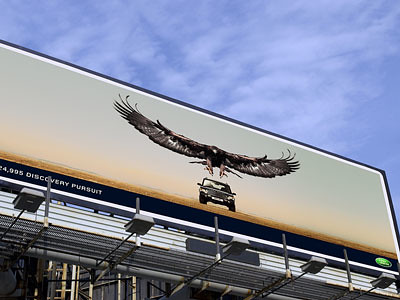The photo captures a close-up view of a prominent billboard advertisement set against a blue sky dotted with puffy white clouds. The billboard is extremely wide and narrow, framed by a white and black border. Dominating the scene is a large eagle with its wings fully spread, reaching halfway across the off-white billboard, its talons appearing poised to grasp the vehicle below. The vehicle is identified as a Land Rover Discovery Pursuit, depicted head-on with its headlights shining. The base of the billboard features a slight brown line representing sand, suggesting a rugged, off-road environment.

In the lower right-hand corner, a green Land Rover logo is placed within a blue bar that extends across the billboard's width. Beside it, in white lettering on a black background, is the text "Discovery Pursuit," with an unreadable number preceding it. The photograph also includes the billboard's supporting silver structure and some elements of surrounding buildings in the lower left, adding depth to the scene.